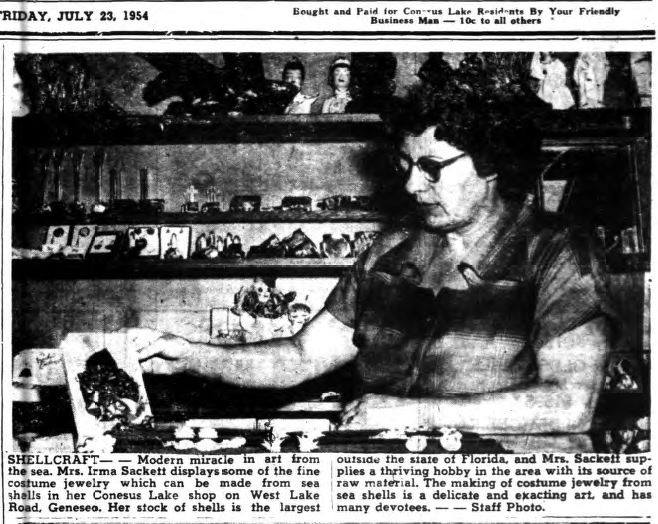This black and white newspaper clipping from Friday, July 23, 1954, features a photograph of Mrs. Irma Sackett in her Kinesis Lake shop on West Lake Road, Genesee. The image, slightly wider than it is tall, captures a middle-aged woman with short, curly hair and glasses, standing centrally in the frame. She is holding up a piece of costume jewelry made from seashells. Surrounding her are shelves filled with various trinkets, dolls, rocks, and numerous shells, highlighting her extensive collection. The caption beneath the photo reads, "Shellcraft, modern miracle in art from the sea. Mrs. Irma Sackett displays some of the fine costume jewelry which can be made from the shells of her Kinesis Lake shop on West Lake Road. Her stock of shells is the largest outside the state of Florida, and Mrs. Sackett supplies a thriving hobby in the area with its source of raw material. The making of costume jewelry from seashells is a delicate and exacting art." The clipping also mentions it was a 'Staff Photo' and notes at the top, "Bought and paid for Kinesis Lake Residence by your friendly businessman, $0.10 to all others."